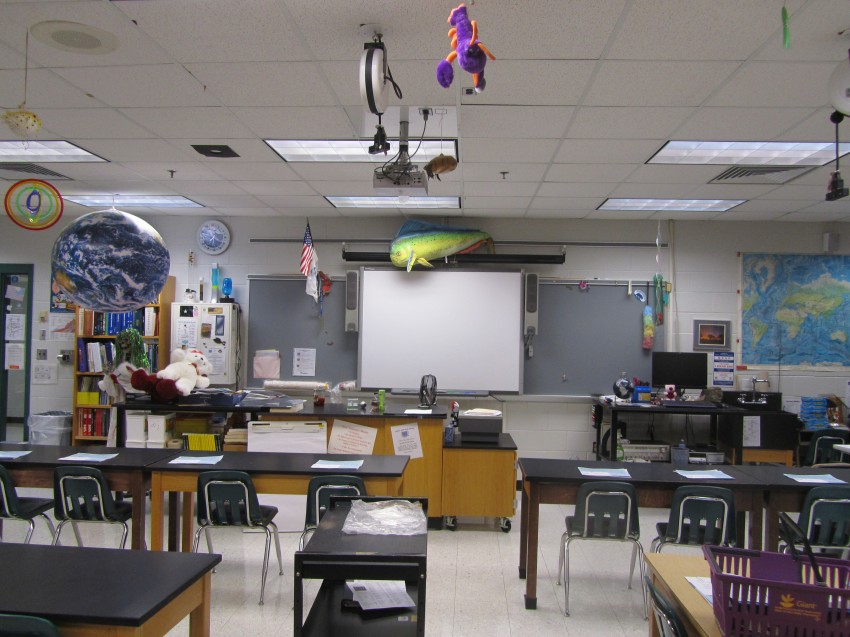This image depicts a bustling American science classroom, possibly for high school or middle school students. The room is filled with a variety of desks and chairs, neatly aligned horizontally to promote a sense of unity. At the front, the teacher’s desk is cluttered with papers and teaching materials, while the whiteboard behind it, flanked by two speakers, serves as a focal point for instruction. Decor elements include a large globe, a skeleton adorned with a wig, and a teddy bear, adding a playful touch to the scientific environment. The ceiling is festooned with hanging decorations such as a stuffed lobster, fish, and puffer fish, enhancing the room’s engaging atmosphere. An American flag proudly hangs on the wall, and books line the shelves, indicating a rich resource area. In addition to a chalkboard and an overhead projector screen, there are notable features like a monitor and a fridge to support both educational and practical needs. The perspective from the back of the room offers a comprehensive view of this well-equipped classroom, illustrating both functionality and an inviting, energetic ambiance.